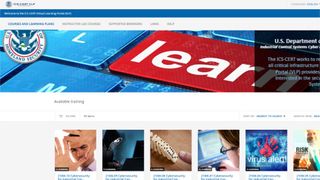Screenshot of a Blurry Website Interface with Key Elements Identified

The screenshot displays a blurred website interface making it challenging to discern specific details. However, visible elements include a horizontal menu bar with five options at the top. Displayed centrally is an American court seal, suggesting a governmental or judicial theme.

Prominently positioned is a red push button labeled 'Learn.' There is a partial, unclear text that hints at it belonging to a department of some sort. Below these main elements, several faint images are visible:

1. A man framing his face with his hands.
2. An individual dressed in black, seemingly engaged in hacking a computer.
3. A close-up of fingers knocking over dominoes.
4. A woman working on a computer.
5. A hand marked in red, reaching across, possibly related to an album or alert named 'Virus Alert.'
6. Text or elements partially indicating something presumably titled 'Risk.'

Overall, the screenshot's low resolution obscures finer details, affecting readability significantly.